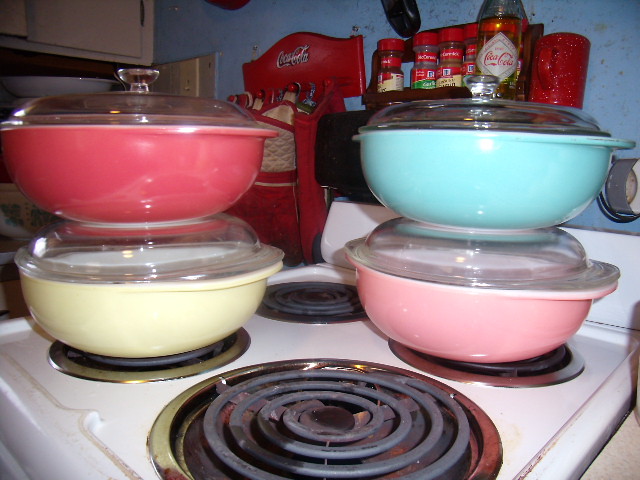The image depicts an older kitchen with a white, coil-burner stovetop. Sitting on the stove are four ceramic containers, each with a glass lid. The containers are colored blue, pink, light yellow, and red, with some stacked on the burners—red on light yellow and blue on pink. The background features a blue wallpaper adorned with gold patterns, an array of McCormick spices in a wooden holder, and a Coca-Cola glass bottle. Additionally, a red mug with white sparkly bits sits next to the spice rack. There is a red Coca-Cola sign with white text and hanging oven mitts nearby. In the top left corner, an old white cabinet is attached to the wall. The kitchen exudes a nostalgic, cluttered ambiance, with some debris visible on the wall.